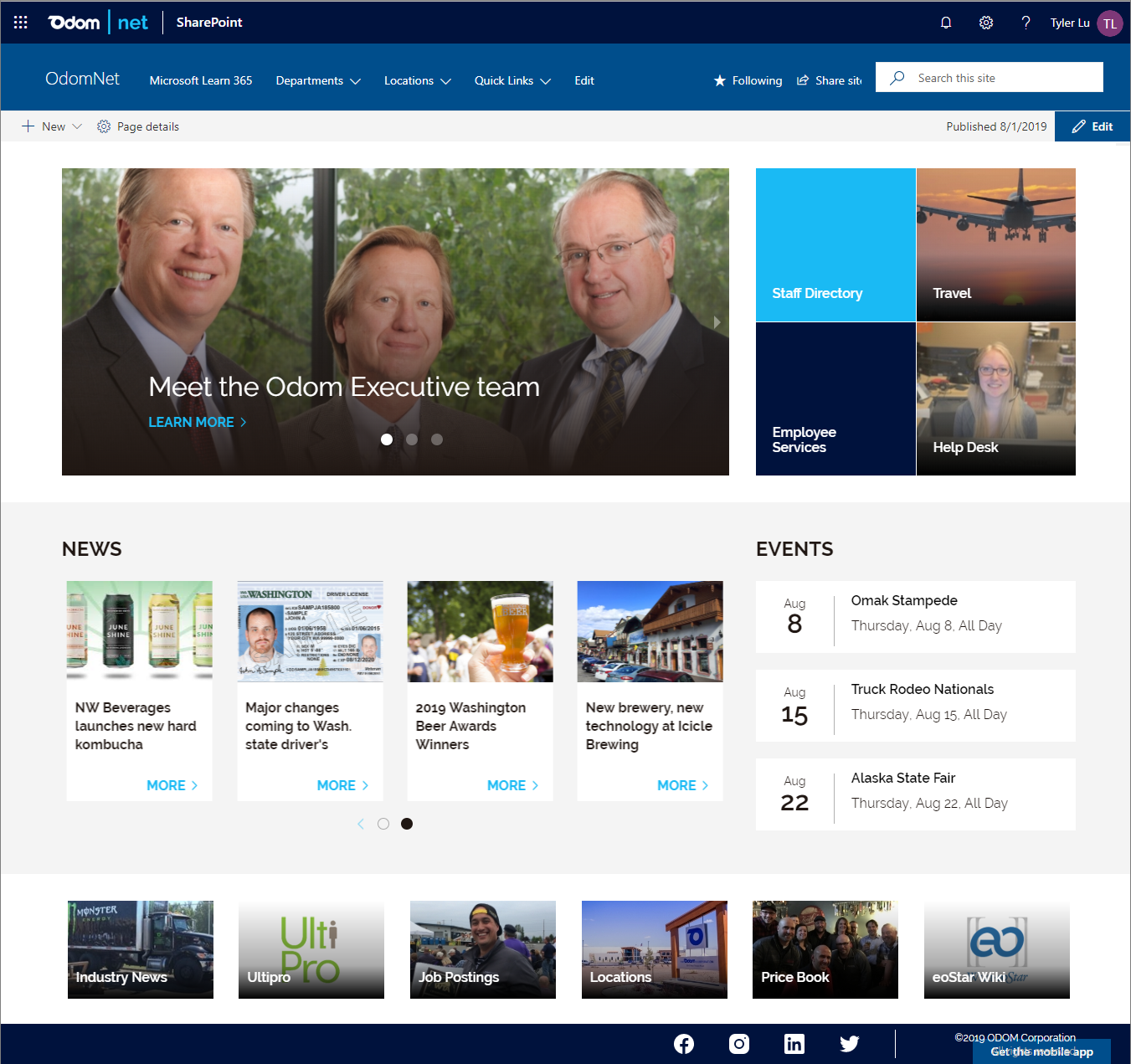This image showcases an organizational SharePoint webpage for Odum, branded as “OdumNet.” At the top of the page, the header features the Odum logo accompanied by the stylized text “net” in blue. Adjacent to this, there are icons for notifications, settings, and a user profile labelled “Tyler Liu” with the initials “TL.”

Below the header, the webpage is divided into several key sections, including:

- **OdumNet**: A general landing section.
- **Microsoft Learn 365**: Links and resources for Microsoft’s learning platform.
- **Departments**: Listing all company departments.
- **Locations**: Information about the company's various locations.
- **Quick Links**: Frequently accessed resources.
- **Edit**: Editing options for page content.

Additionally, there are sections for “Following” and a “Share Site” button. A search bar with the placeholder “search this site” and a blue magnifying glass icon is prominently positioned for ease of navigation. The page also notes a “publish date” of August 1, 2019, and features a blue “Edit” button for content modifications.

The main body of the page introduces the Odum Executive Team with a headline “meet the Odum executive team” and a blue “Learn More” button to explore further details. Various sections are dedicated to:

- **Staff Directory**
- **Travel**
- **Employee Services**
- **Help Desk**

In the news section, the following articles are listed:

1. **NW Beverages Launches New Hard Kombucha**: Featuring images of the new “Jungle Shine” kombucha cans.
2. **Major Changes Come to Washington State Drivers**: Highlighting changes with an image of a Washington State Driver's license.
3. **2019 Washington Beer Awards Winners**: Accompanied by an image of a glass of beer.
4. **New Brewery, New Technology at Icicle Brewing**: Showcasing the exterior of a new brewery building.

The events section and a variety of tabs are located at the bottom of the page, along with social media icons for Facebook, Instagram, Indeed, and Twitter, enhancing connectivity and information sharing.

The overall design of the webpage predominantly features a white background accented with blue borders, ensuring a clean and professional aesthetic.